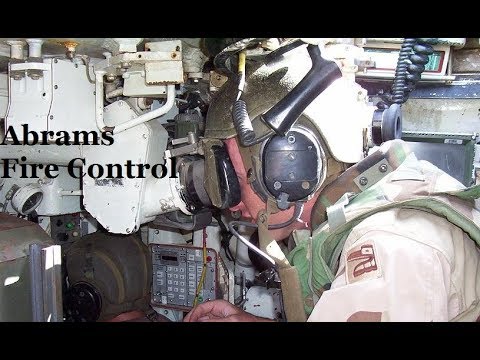The image appears to be set inside a military vehicle, likely a tank or a submarine, and prominently features the text "Abrams Fire Control." The photo captures a soldier in a very cramped, taupe-colored space, indicative of military operations. The soldier wears a green helmet and large earphones, and you can see a side view of his face, revealing only his eye, part of his nose, chin, and mouth. He is intently looking into a white spectroscope or telescopic device, with a black peephole. His uniform consists of a white shirt adorned with two reddish-brown designs resembling shoes on the shoulder, over which he wears a green army vest. The background is cluttered with wires, metal components, and a computer with numerical displays. Directly in front of him, there is a small keyboard, and below the white contraption he's focused on, the back of another soldier's head—also in a green helmet and black earphones—is visible. The overall atmosphere suggests a high-stakes environment where precision and focus are critical.